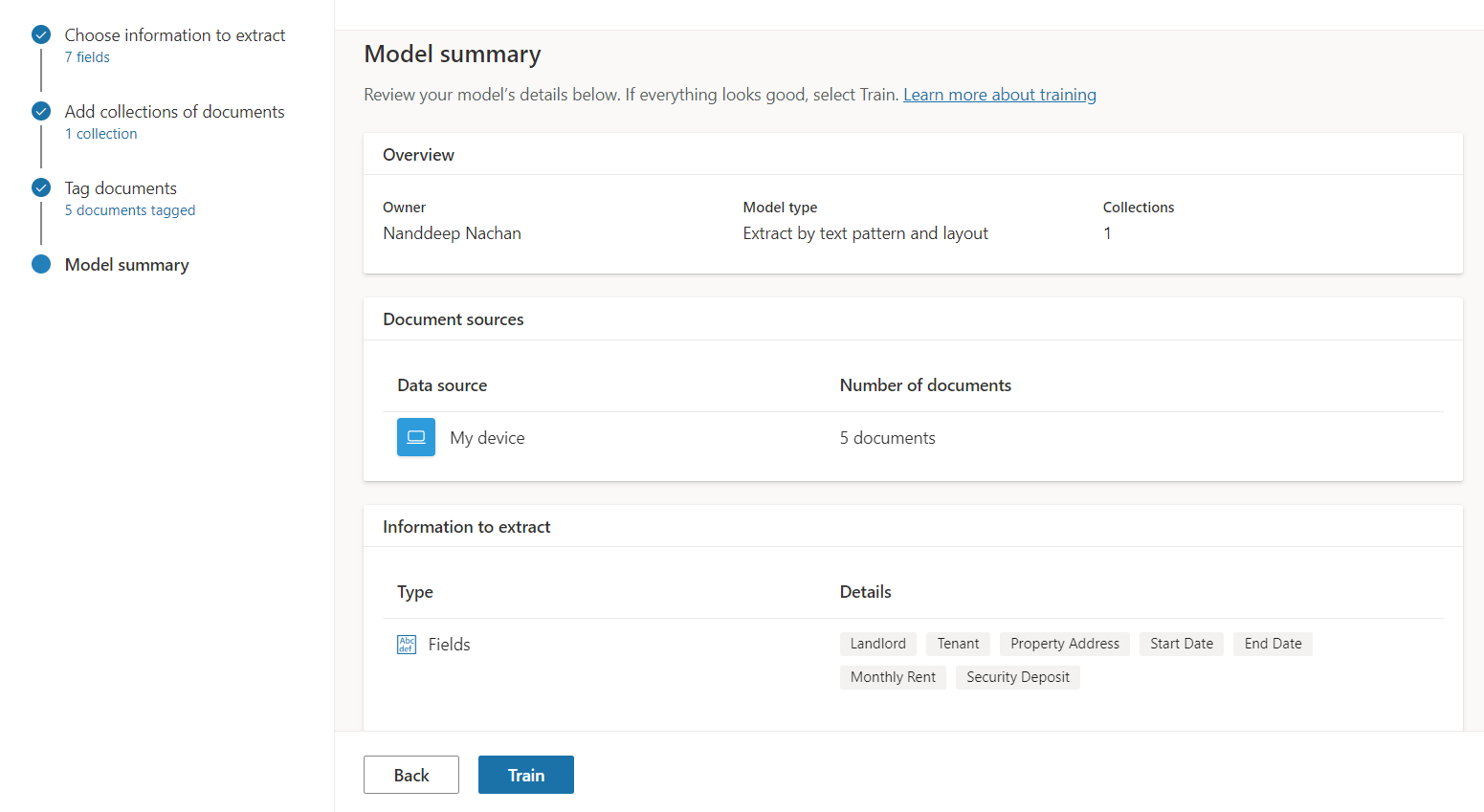The image displays a webpage titled "Model Summary." It serves as a review screen for a machine learning model or AI project, outlining specifics before initiating the training process. The model appears to focus on extracting information patterns from text, particularly concerning real estate and housing documents. Key details include:

- **Owner:** Nandeep Nakan
- **Model Type:** Extract by Text Pattern
- **Layout Collections:** One
- **Document Sources:** Data Source - My Device
- **Number of Documents:** Five

The information to be extracted comprises various fields: Landlord, Tenant, Property Address, Start Date, End Date, Monthly Rent, and Security Deposit. 

On the left side of the page, a navigation pane highlights the steps already completed, including "Choose Information to Extract" and "Add Collections Documents." The current view is the final step, summarizing the progress made.

At the bottom of the page, there are navigation buttons: a 'Back' button and a blue 'Train' button, indicating that the user is ready to proceed with training the model.